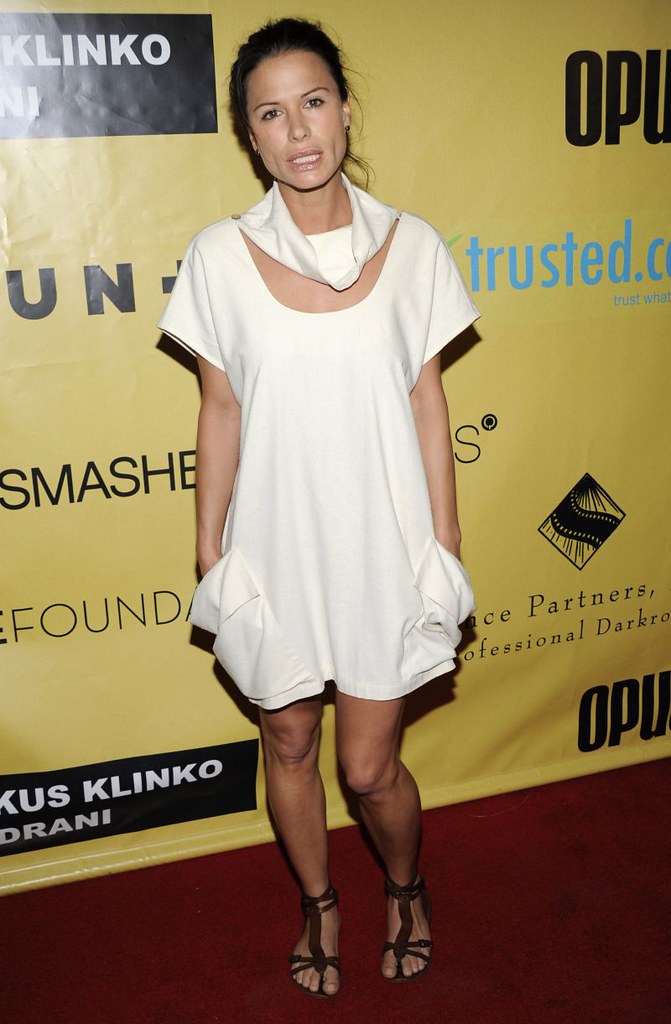In the image, a woman who appears to be a famous actor stands on a dark red-brown carpet. She has dark hair pulled back and wears a short off-white dress with a low scoop neck and oversized pockets. Around her neck, she has a white scarf, and she is wearing high heel sandals. Her expression is a semi-smile or talking gesture, with her mouth slightly open. The background features a yellow canopy with various brand names and words in black, blue, and white letters, including "Trusted," "Klinko," and "Professional Darkroom." Additionally, there is a black diamond with a filmstrip design on it. The overall scene is somewhat dark, but the woman stands out with her distinctive attire and presence on the red carpet.